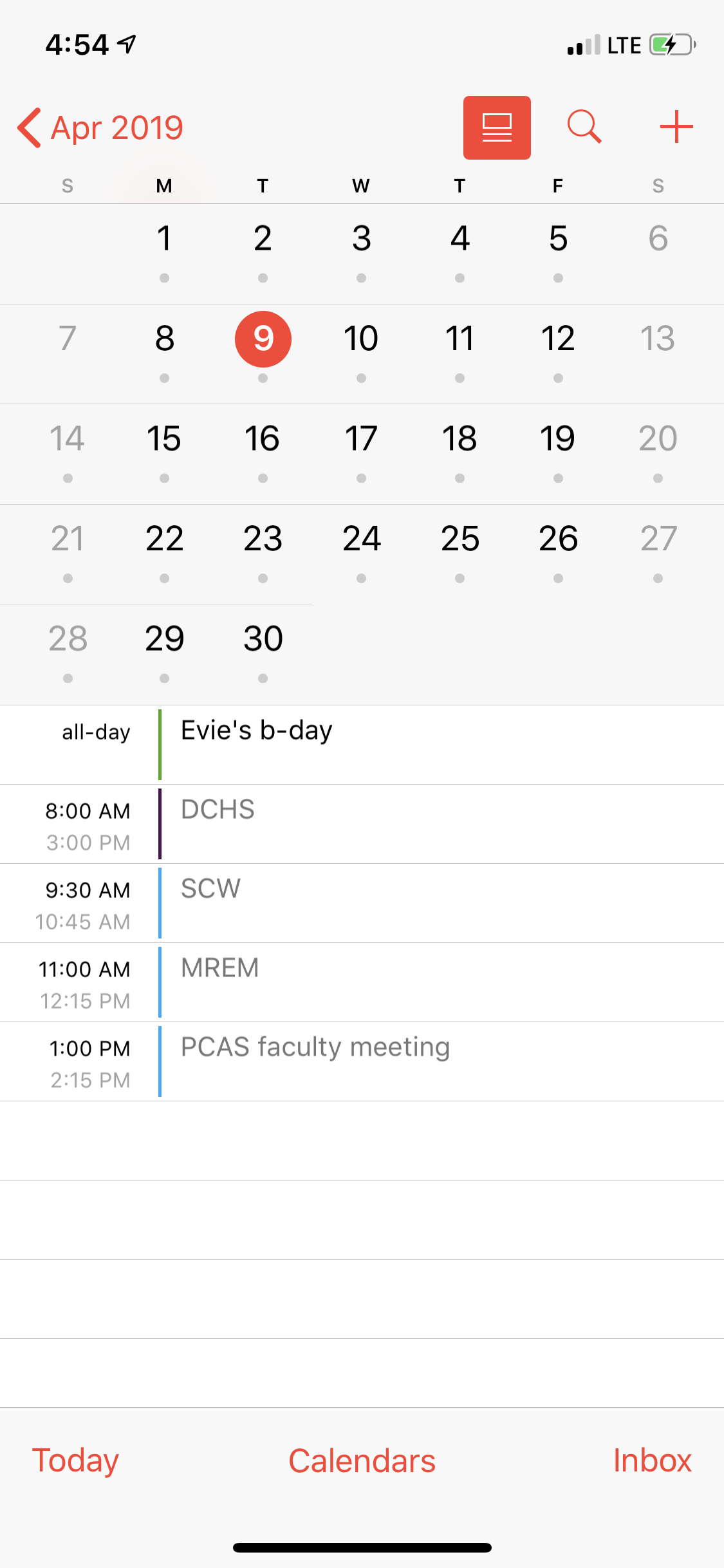Screenshot of a cell phone displaying a calendar for April 2019. The image has a light gray background and is taller than it is wide. In the upper left corner, the time is displayed as 4:54 in black text. The upper right corner shows the phone's signal strength, LTE connectivity, and a battery indicator that is approximately half charged, indicated by green color.

The calendar at the top is set to a month view. The month starts on a Monday, April 1st, and ends on a Tuesday, April 30th. There are five rows of dates, and April 9th is highlighted with a red circle around the date, indicating it is the current day (April 9th, 2019).

Below the calendar, the user's schedule is listed for the day:

- All day: EV's B-Day
- 8:00 a.m.: DCHS
- 9:30 a.m.: SCW
- 11:00 a.m.: MREM
- 1:00 p.m.: PCAS Faculty Meeting

The detailed schedule suggests that the phone's owner might be an academic, potentially a college professor.

At the bottom of the screen, a gray rectangular menu bar is visible with the options "Today," "Calendars," and "Inbox" displayed in red font. The "Calendars" option is underlined in black, indicating it is currently selected, as confirmed by the visible monthly calendar above.